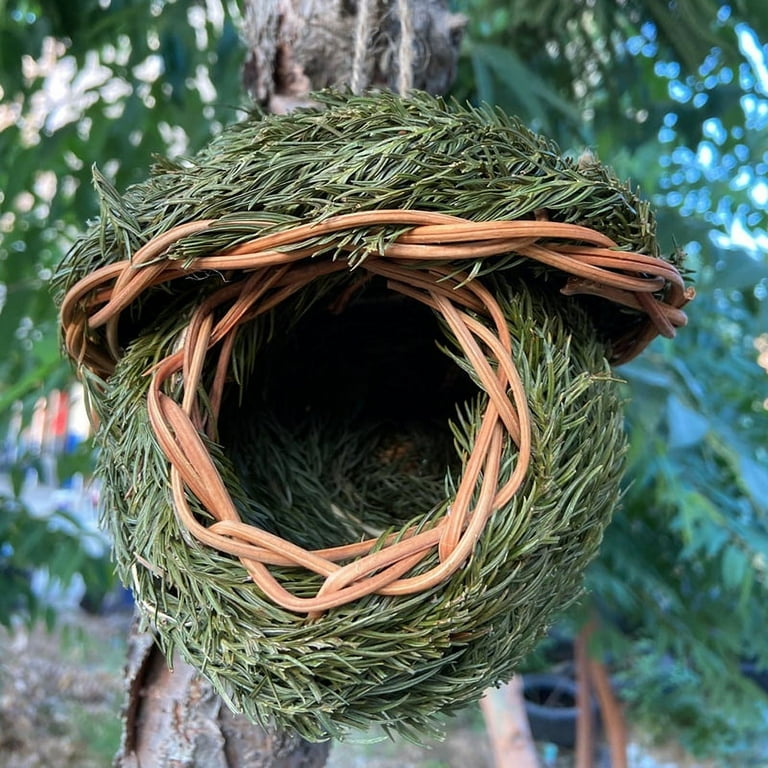This outdoor photograph features an exceptionally crafted and artistic birdhouse mounted on the trunk of an old gray and brown tree. Nestled amidst the blurred backdrop of green leaves and blue sky, the birdhouse stands out with its intricate, natural appearance. It is meticulously made from materials resembling pine needles and fir branches, creating a rounded, hollow ball with a circular entrance hole in the center. This entrance is framed by twisted wood, giving it a cozy and inviting look. The top of the birdhouse is adorned with an upside-down shallow bowl-like structure crafted from the same green material, enhancing its artistic charm. The combination of these natural elements and the thoughtful design makes it a unique and perfect home for a lucky bird.